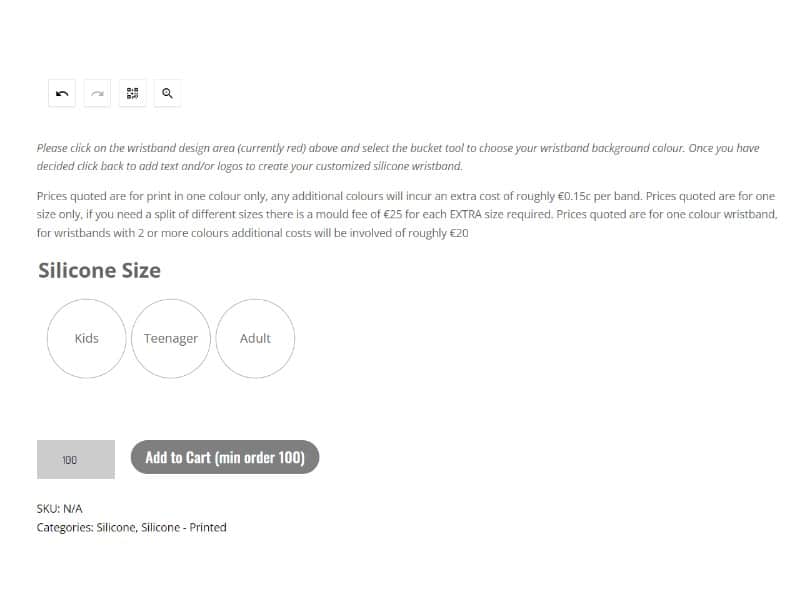The image portrays a website interface dedicated to the customization of silicone wristbands. At the center of the screen, a message instructs users to click on the currently red wristband design area and utilize the bucket tool to select a background color of their choice. After choosing a background color, users are directed to click back in order to add text and/or logos to create their custom wristband.

Pricing information is prominently displayed, noting that the quoted prices encompass single-color prints only. Each additional print color incurs an extra cost of approximately 15 cents per band or £15. The prices are specific to one wristband size; requesting multiple sizes triggers a mold fee of £25 for each additional size. Furthermore, wristbands with two or more colors will involve additional costs, estimated at about £20.

The wristband sizes available for customization include options for kids, teenagers, and adults. There's an interactive feature for users to specify the quantity, with a minimum order requirement of 100 units clearly indicated beside the "Add to Cart" button. The SKU and category information—listed as silicone and silicone printed—are found in the product description area.

At the top of the page, navigation aids such as a back arrow and a magnifying glass icon are visible, allowing users to navigate through the site and search for other products. Overall, the website offers a streamlined process for creating personalized silicone wristbands, with detailed information on customization options and associated costs.